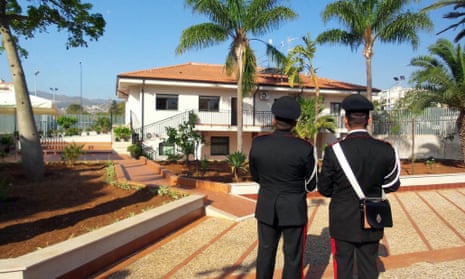The photograph showcases two men dressed in black, somewhat floppy hats, and black uniforms with red stripes down their pants. One of the men carries a pack over his shoulder. They are positioned slightly off-center towards the bottom of the image, standing side by side with their backs to the viewer. They stand on a walking path in a courtyard made of beige stone with inlaid red bricks. The men are facing a two-story white house with a brown roof, which features a balcony. Surrounding the house are several palm trees, one prominently to the far left. To the left of the house lies a pool. The backdrop of the scene is a clear, bright blue sky with no visible clouds, enhancing the vivid colors of the setting. The overall atmosphere suggests a military base due to the men's uniforms and stance.